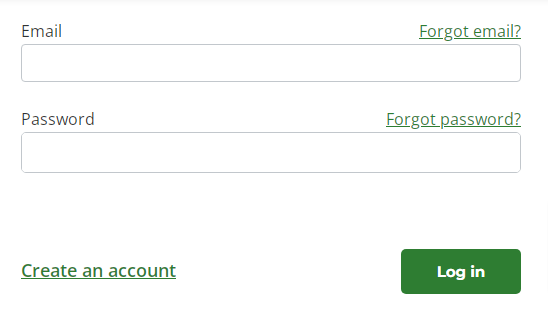The image depicts a login interface with fields and options for user authentication. At the top, there is a text link on the far right underlined with "Forgot email?" for users who may need to recover their email information. Below this link, there is a rectangular input field labeled "Email," where users can type their email addresses. Directly beneath the email entry, there's another link, "Forgot password?" in green text, helpful for users who need to reset their passwords.

Following this, there's a password input field designed similarly to the email field, where users can type in their passwords. Positioned at the lower right-hand corner of the interface, there is a green rectangular button with curved edges, featuring the text "Log in" in white print for users to proceed with authentication.

In the bottom left-hand corner of the image, there is a green underlined link labeled "Create an account" for new users who need to set up a login. The overall design is clean and user-friendly, offering both login and account creation functionalities along with assistance for email and password retrieval.